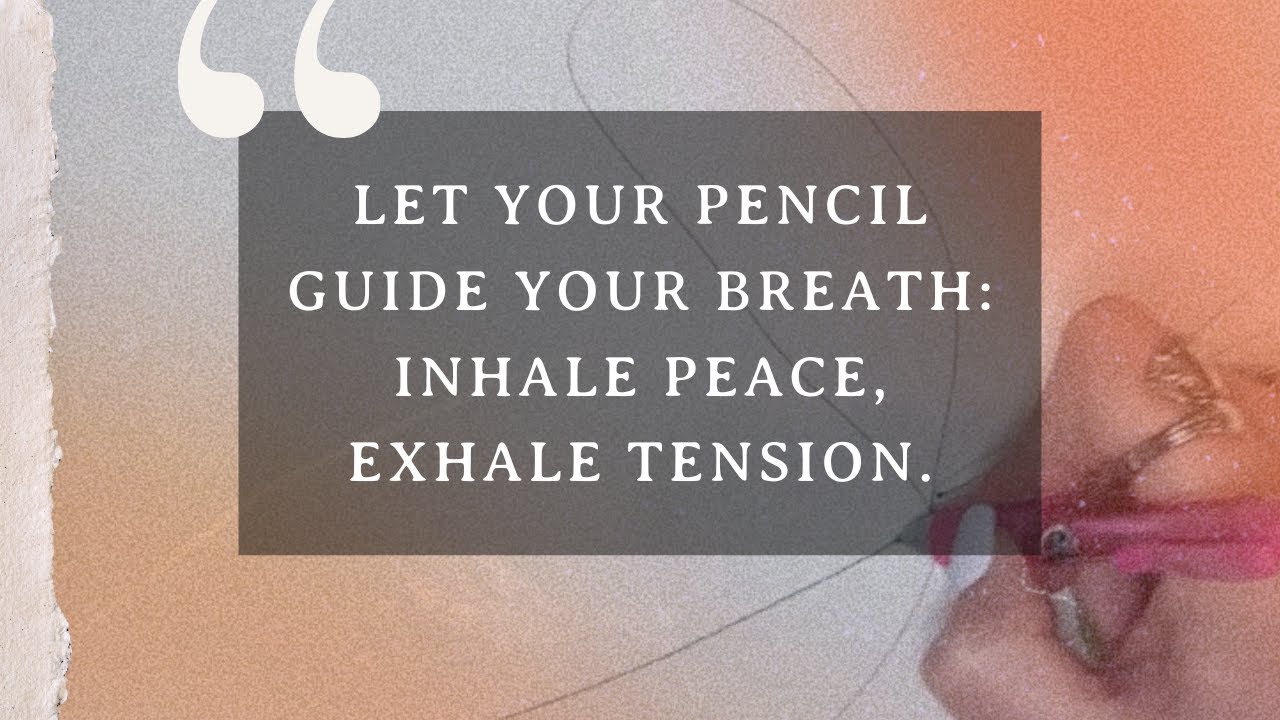The image portrays a detailed scene with multiple elements. At the top, a peach-colored banner with black text reads "Calm Yourself," underlined, followed by "with breathwork + doodling." Below this, a thin orange strip with white hand-marked Xs adds subtle texture to the composition. The central focus is on a hand sketching in a spiral-bound sketchbook, using a dark pink mechanical pencil. The hand, adorned with a ring on the forefinger, features a thumb painted with white nail polish. To the right of the sketchbook, there are twelve circular color samples arranged in three rows. Each row showcases different hues: the top row is pink, followed by yellow, purple, and a deep turquoise, demonstrating the variety of colors available with the pens. The overall backdrop includes a mix of patterned sections and solid colors, adding depth to the visual appeal.